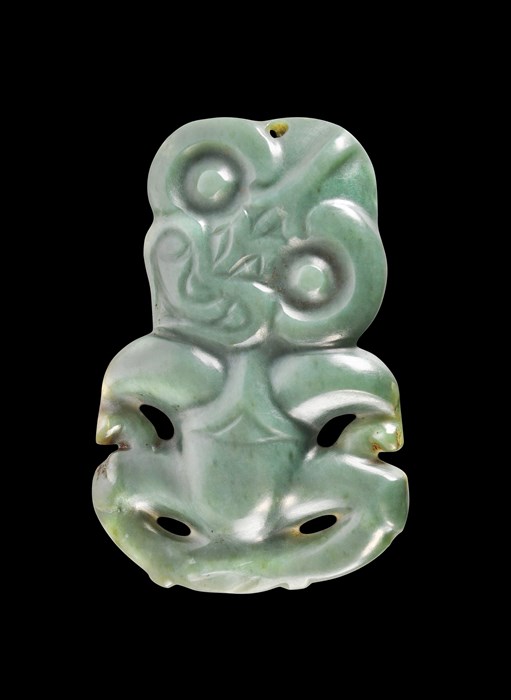The image features a zoomed-in photograph of a meticulously crafted jade amulet against a solid black background, creating the surreal effect of the amulet floating in a void. The amulet, made from lustrous green jade, depicts a whimsical creature characterized by a round head slightly tilted to the right. The face of the creature is adorned with a large, toothy smile complete with fangs, and it has small, indented eyes that add to its playful yet mysterious appearance. The body of the creature is also round, with its arms and legs curving inward towards itself, giving it a compact and endearing form. The polished surface of the jade catches light, casting subtle highlights and adding depth to the intricate carving. There is a hole at the top of the amulet, suggesting it is intended to be worn as a pendant. The black background enhances the polished green of the jade, making the details of the creature's form stand out vividly. The overall aesthetic makes the amulet appear almost otherworldly, accentuated by the focused lighting coming from the right side, which further highlights its sculptural features.